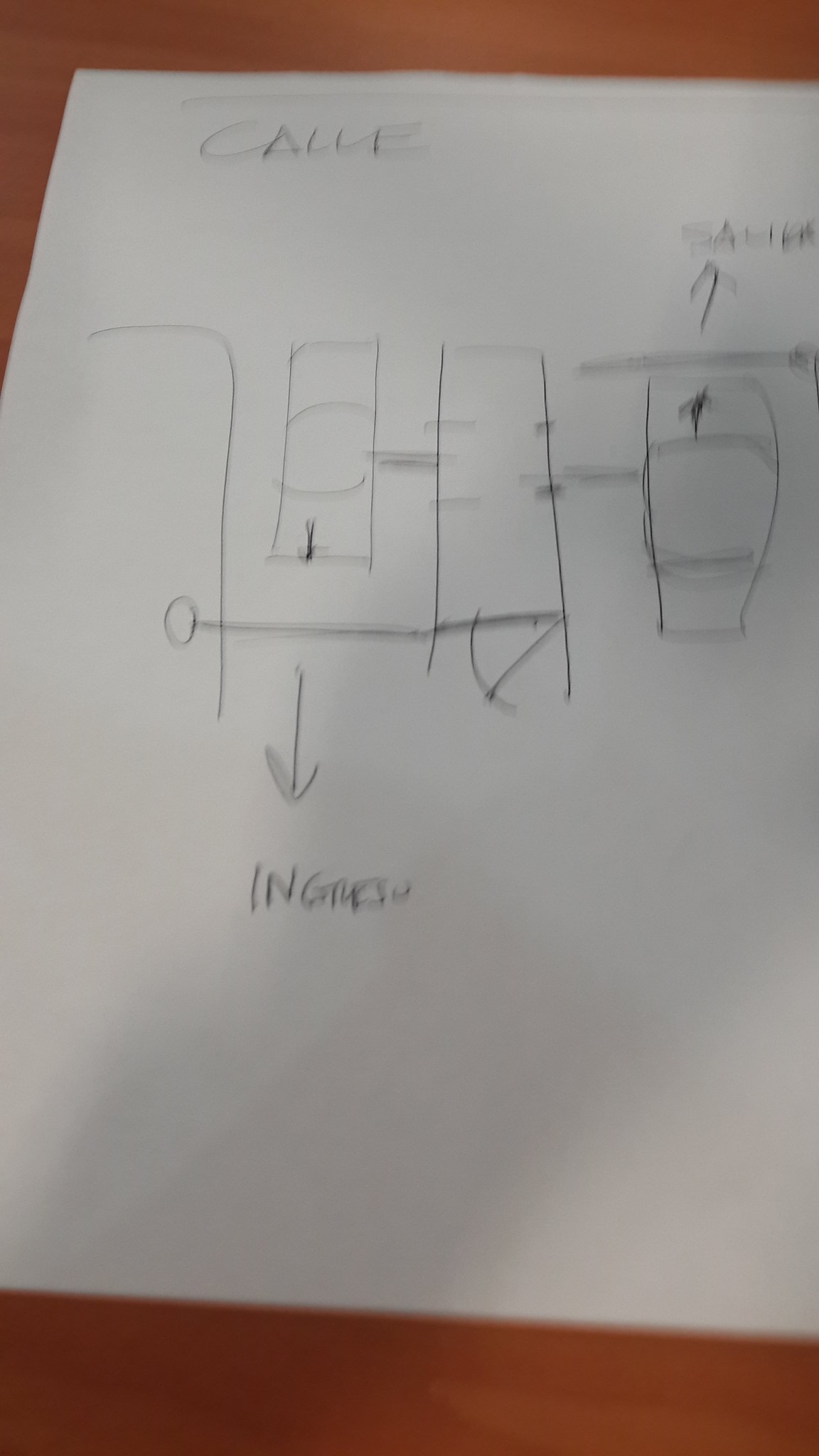A hand-drawn illustration in black biro pen, captured with a low-quality smartphone camera, resulting in a slightly blurred and grainy image. The white sheet of paper displays faint pink and green tones, particularly near the bottom, with an array of tiny dots forming the intricate sketch. The paper is not perfectly centered in the frame, revealing the wooden surface background along the bottom, left side, and top edge. Oriented in portrait, the drawing includes faint, handwritten words: "INGR" followed by indistinct letters at the bottom, and a partially visible "SALIA" near the top right corner. The illustration, titled "Calle" at the top, depicts a top-down diagram featuring rectangular shapes resembling vehicles in portrait orientation. Additional elements include directional arrows, one leading downwards to "ING" and another upwards to the "SAL" word, intersecting lines, and an upside-down, backward capital "L" on the left. The text labels do not appear to be in English.